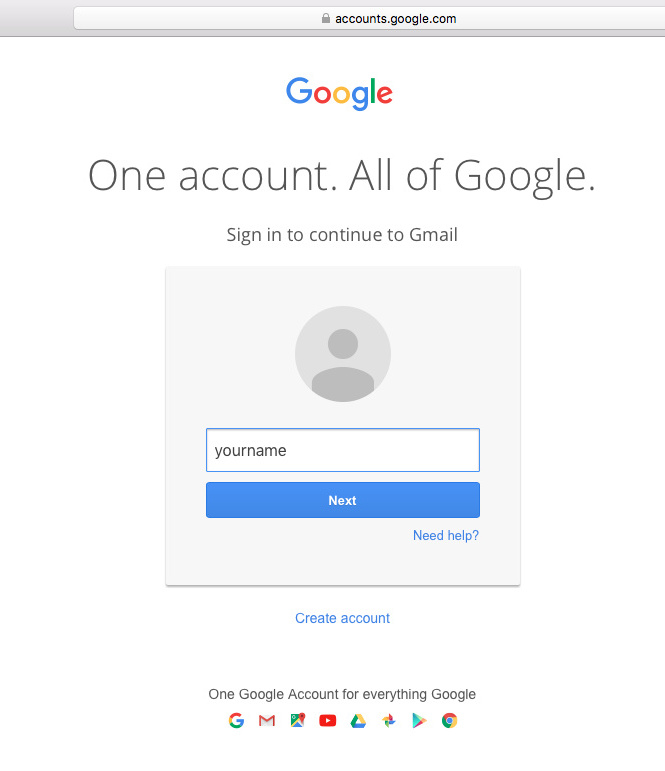Here is a detailed and cleaned-up descriptive caption for the image:

---

The image is a screenshot of the Google sign-in page, set against a clean, white background. At the very top, there's a faint gray border, above which the web address "accounts.google.com" is displayed in darker gray font on a light gray backdrop. To the left of the web address, a small padlock icon indicates that the website is secure.

In the center of the page, the iconic Google logo is prominently featured. The logo spells out "Google" with a capital blue "G", followed by red, yellow, and blue "o"s, a green "l", and a red "e". Just below the logo, a medium-sized font states: "One account. All of Google." Underneath this, in a smaller font, the message: "Sign in to continue to Gmail" is clearly written.

A centrally aligned light gray box is present beneath this text, which contains a dark gray circle icon symbolizing a user account without a profile picture. Inside the box, there's a rectangular field labeled "Your name" where the user would enter their username. Below this field is a blue rectangle with white text that reads "Next," which users click to proceed.

Adjacent to the "Next" button, on the right side, a blue hyperlink reads "Need help?" with a question mark, indicating assistance is available. Just below the user icon and back on the white background, another blue hyperlink labeled "Create account" invites new users to register for a Google account.

At the very bottom of the page, a line of text in gray font declares: "One Google Account for everything Google," followed by an array of small icons representing various Google services, including the Google search engine, Gmail, Google Maps, YouTube, Google Drive, Google Photos, Google Play, and the Chrome browser.

---

This descriptive caption comprehensively details the visual components and the layout of the Google sign-in page.